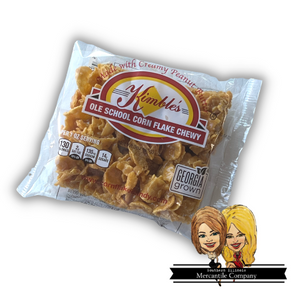This image showcases an advertisement for "Kimball's Old School Corn Flake Chewy," a food bar made with creamy peanut butter. The bar is displayed tilted slightly to the right on a white background. It is packaged in a clear plastic bag with a grey outline. The packaging prominently features nutritional information, specifying 130 calories. There is a "Georgia Grown" symbol indicating it is produced in Georgia. In the lower right corner, the packaging displays an image of two women— one with shoulder-length brown hair and the other with long blonde hair. These women appear to be associated with the product. Additionally, a black banner with partially visible writing indicating a company name is also present.